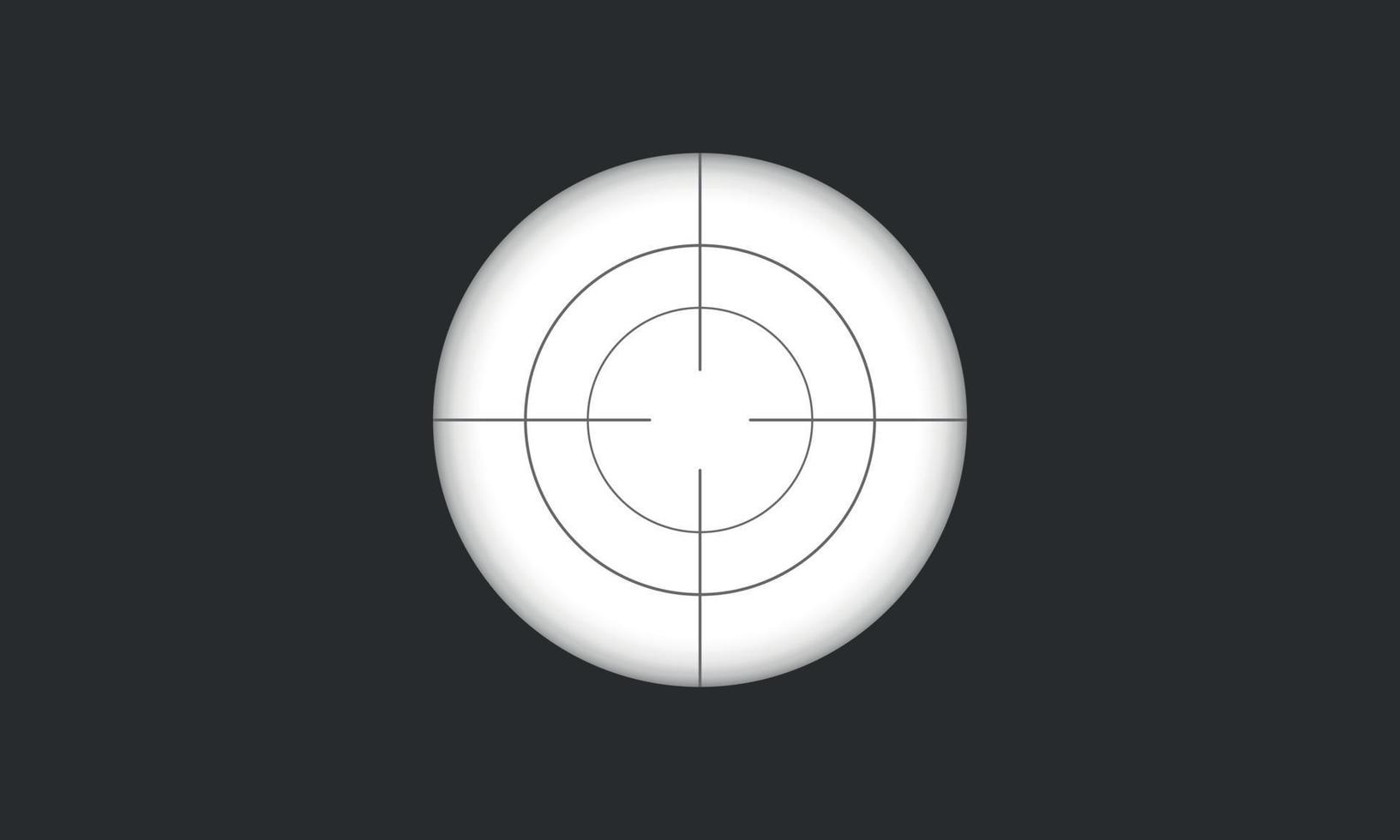The image features a horizontal, landscape-oriented rectangle with a solid, featureless dark blue or navy blue background. Dominating the center is a white circle whose diameter spans roughly a third of the frame's length. This circle contains a detailed target pattern, characterized by thin black lines forming a mandala-like design. Four straight lines, positioned at right angles, radiate from a small, central void, extending toward the perimeter where they intersect two concentric black rings. Surrounding the circumference of the white circle are two thin, blurry gray borders, with the outer one appearing darker than the inner one. The overall composition evokes the look of a glowing periscope viewfinder or a stylized eye, centered against the starkly contrasting dark background.